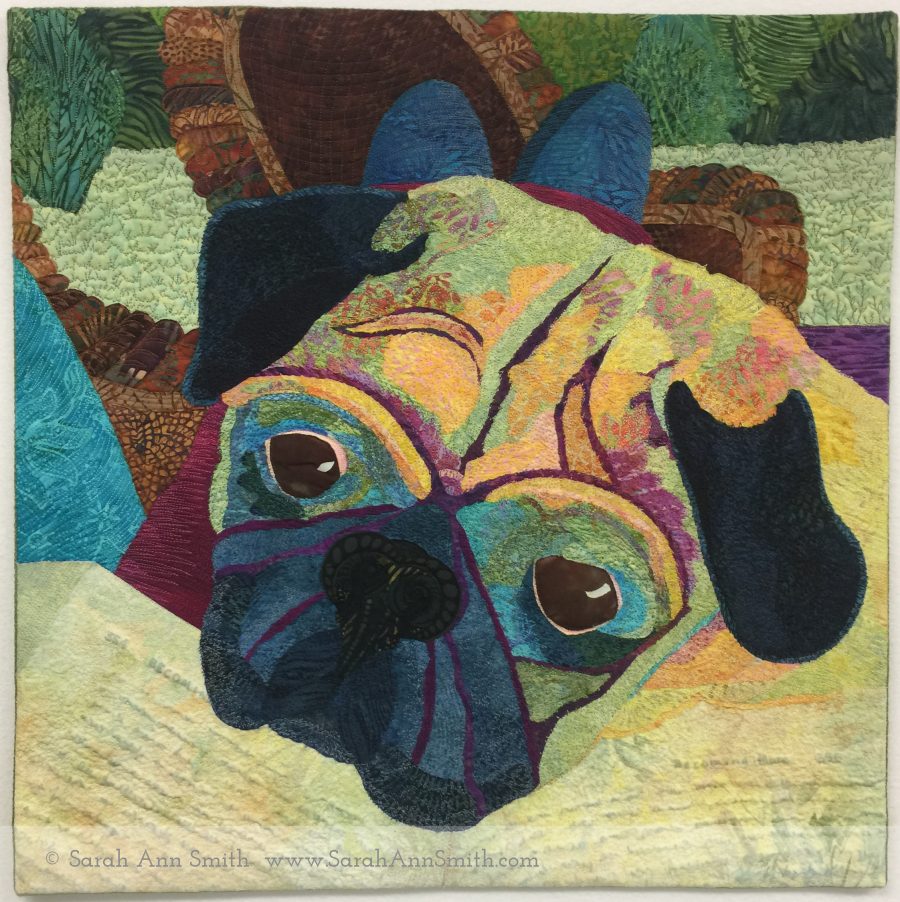This detailed artwork features a close-up of a pug's face, vividly brought to life through various hues and textured patterns that give the impression of a fabric-based composition. The pug's droopy black ears frame a face richly adorned with colors and intricate details. Striking wrinkles cover the dog's visage, enhanced with shades of pink around the forehead and detailed lines near the eyes, which are meticulously colored in greens and blues, encircling its expressive brown eyes. The jowls are shaded with dark blue tones, adding depth and prominence to the facial features. Swirling dots and elaborate lines around the nose contribute to the piece's intricate look. The dog's head appears to be resting on a surface, enhancing the close-up effect, with the background featuring varied textures that complement the main subject's vibrant palette. At the bottom of this colorful and texture-rich masterpiece, a watermark reads "Copyright Sarah Ann Smith, lew.sarahannsmith.com," acknowledging the artist's unique creation.